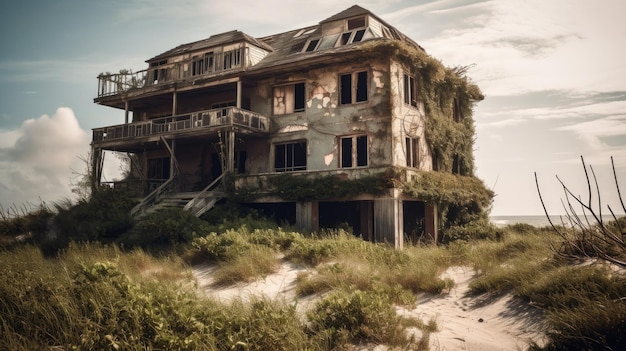The image depicts a deteriorating, multi-story mansion-like house situated on a beach. The house, which appears to be on stilts, is covered in peeling plaster, revealing patches of pink beneath its grey exterior. Moss, vines, and greenery have aggressively taken over much of the structure, especially on the left side. The windows are devoid of glass, adding to the sense of abandonment, and the two precarious balconies—on both the second and top floors—seem ready to collapse. The mansion's once broad and impressive front door is now accessed by steps that lead to nowhere, with no visible driveway in sight. In the foreground, the sandy beach is dotted with clumps of brown and green grass and brush. The backdrop features a dynamic sky, with varying shades of white, grey, and blue clouds hinting at an approaching storm. Just behind the house, a glimmer of water peeks through, reinforcing the location's proximity to the ocean. Despite its current state of decay, the structure hints at the grandeur it must have once possessed.